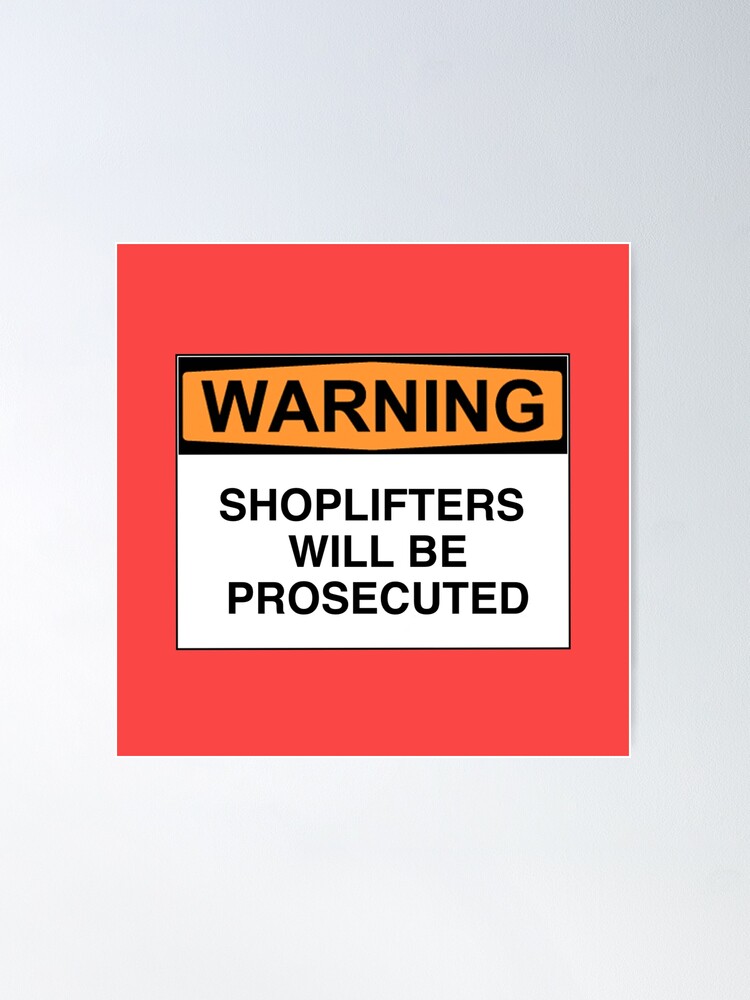This image depicts a vibrant graphic design of a warning sign, presumably created digitally. The central focus is a bright pink square bordered by a thin white outline, giving it a framed appearance as if mounted on a light gray, possibly textured wall. The pink background is striking and vibrant, with two key sections of text. 

The top section features the word “WARNING” in bold, uppercase black letters against a bright burnt orange rectangle, highlighted with a black outline. Below, in a white rectangular section, the text “SHOPLIFTERS WILL BE PROSECUTED” is similarly rendered in a bold, uppercase black font, resembling the Helvetica typeface. The entire composition appears to employ shadows and details that suggest the use of Photoshop, enhancing the digital and artistic quality of the warning sign.